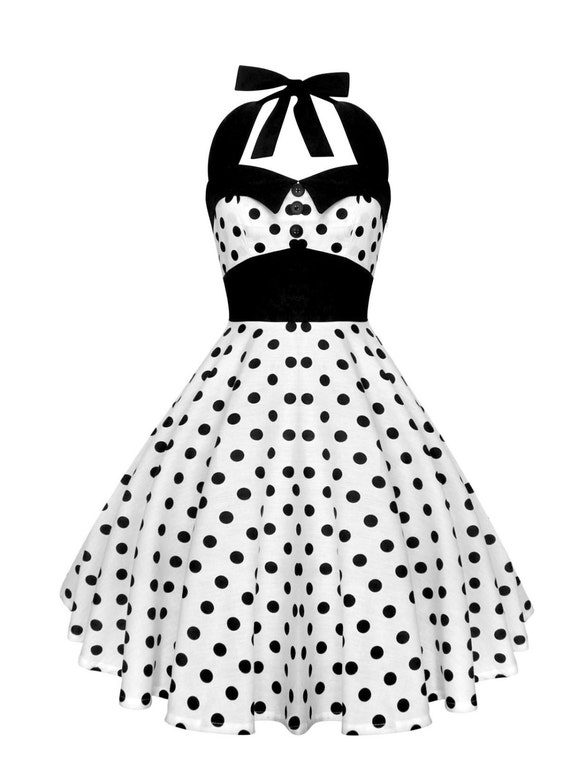This image features a charming 1950s-style black and white polka dot dress, seemingly suspended against a plain white background as if floating. The dress has a halter neck design with two black straps that tie behind the neck, and a black collar that accentuates the neckline. The bodice is white with black polka dots and includes a front placket with four buttons. The waistline is cinched by a broad black band, creating a flattering silhouette. The skirt is also white with black polka dots, flaring out below the waist in soft pleats that add a touch of elegance and movement to the dress. The attention to detail and vintage-inspired design make this dress both adorable and stylish.